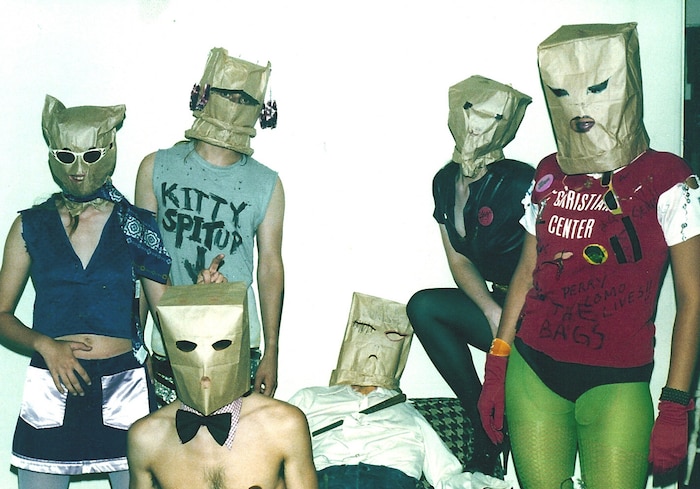This photograph features a group of six individuals who appear to be dressed in an eclectic and possibly punk-inspired fashion, reminiscent of a band from the 70s or 80s. Each person has a paper bag over their head, with cut-outs for the eyes and mouth, and various unique decorations on the bags. Starting from the right, one individual is wearing green tights, black bottoms, and a red t-shirt that has "The Bags" written on it in marker. Next to them is a female figure in a black shirt with a pink button, black tights, and another person in red gloves. Centrally on a sofa is a man seemingly passed out or leaning back, dressed in a white business shirt and blue jeans. Crouched down is a shirtless man with a black bow tie and another bag on his head. Behind him is a person in a blue t-shirt that says "Kitty Spit Up" with an arrow pointing downward, and finally, an individual can be seen in a skirt and blue top. The image is quirky and odd, suggesting a theme party or a band promotional shoot, where the detailed costumes and bag masks with added faces create a bizarre and captivating visual.